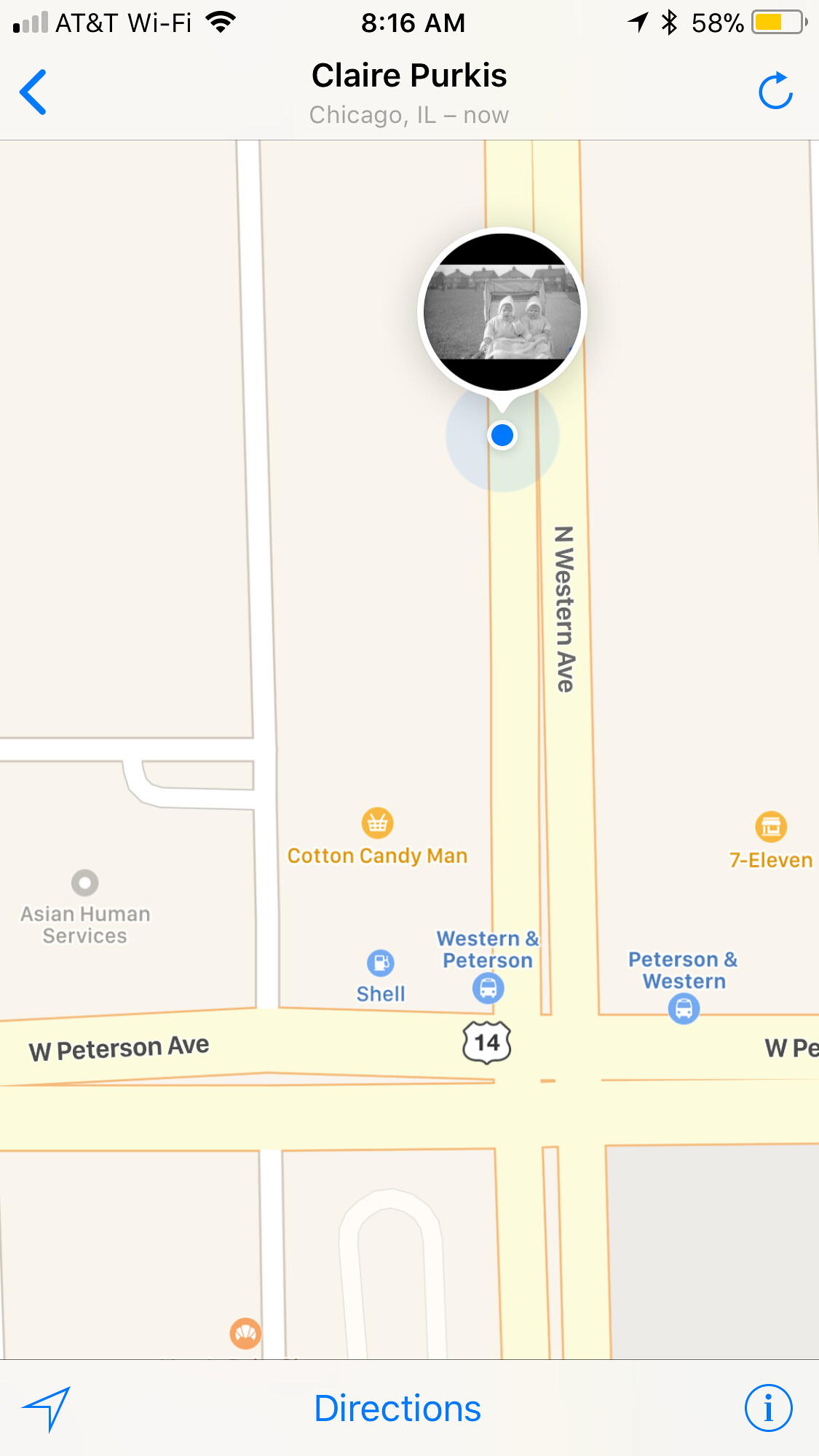This screenshot from a smartphone, displaying the Google Maps interface or a GPS application, depicts a location in Chicago, Illinois. The top of the screen shows the name "Claire Perkis" and the current time of 8:16 a.m. The phone's battery is at 58% and is connected to AT&T Wi-Fi with only one signal bar. The map centers on Northwestern Avenue, indicated by a small blue dot representing the user's location. Above this dot is a small, black and white profile photo of two people, which is difficult to see clearly.

Northwestern Avenue intersects with West Peterson Avenue, and prominent landmarks include a Shell gas station on the corner of Northwestern and Peterson, and a 7-Eleven on the opposite side of the street. Nearby businesses include Asian Human Services and the intriguingly named "Cotton Candy Man." At the bottom of the screen, the word "Directions" is visible, suggesting the user may be navigating somewhere.